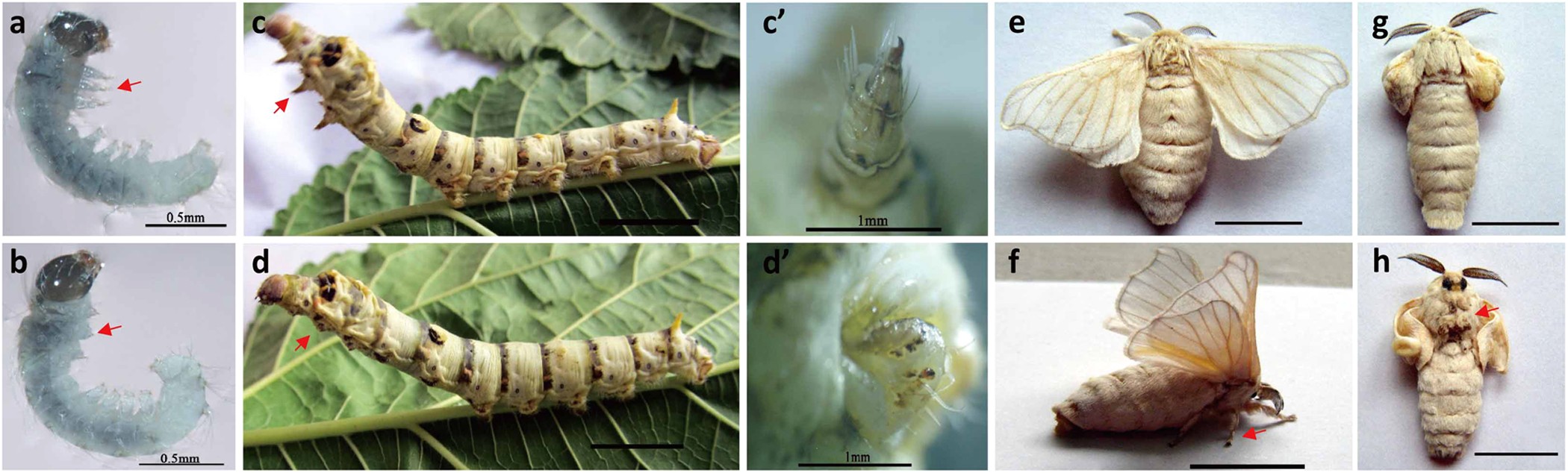The image displays a detailed depiction of the lifecycle of a caterpillar transforming into a moth, arranged in a ten-panel grid format. Each panel represents a different stage in the metamorphosis, labeled in black font at the top left with letters A through H, including C' and D'. 

On the far left, panels A and B showcase newly hatched caterpillars with bluish-white bodies and black heads. The small, shrimp-like larvae are depicted with numerous legs and a slight curl, resembling tiny bananas. 

Panels C and D illustrate the intermediate caterpillar stage, where the caterpillars have elongated, taking on a green hue with distinctive black stripes dividing their body segments. A red arrow in panel C points to one of their many legs. The caterpillars are seen walking along the central vein of a rugged leaf.

Transitioning into the chrysalis phase, panels C' and D' feature the caterpillars beginning their pupation. These segments show the caterpillars’ bodies transforming into a more rigid, cocoon-like state, with a whitish coloration and small black dots scattered on their surface.

Panels E and F depict the emergence of the adult moths. In panel E, the moths are fully developed with expanded wings, displaying a white, slightly transparent appearance, with thick, fluffy bodies and moon-shaped black antennae. Their thoraxes appear rotund and adorned with fine fur.

Finally, panels G and H present the moths post-emergence with their wings retracted. These images offer views from different angles—one showing the back and the other the front of the moths. The moths maintain their white, fluffy appearance, although they appear less rotund compared to those in panel E.

The bottom row mirrors the top, again labeled B, D, F, and H, with measurements highlighting the length development at each stage, set against a clean, white laboratory background.